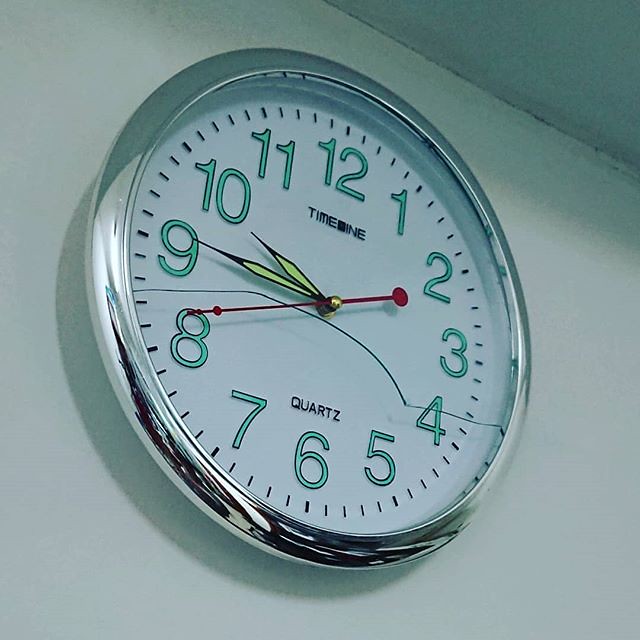A prominently positioned clock adorns a plain white wall. Encased in a sleek chrome silver frame, the clock's design features a pristine white background with bold, turquoise numbers. The clock's hands are frozen at a quarter to ten. The clock face is protected by a glass cover, which reveals a pronounced crack running across its surface, adding an intriguing imperfection to the scene. Emblazoned with the words "Time Nine" at the top and "Quartz" at the bottom, the clock captures a moment in time with striking simplicity. The photograph, unembellished and unprofessional, captures the essence of everyday domesticity.